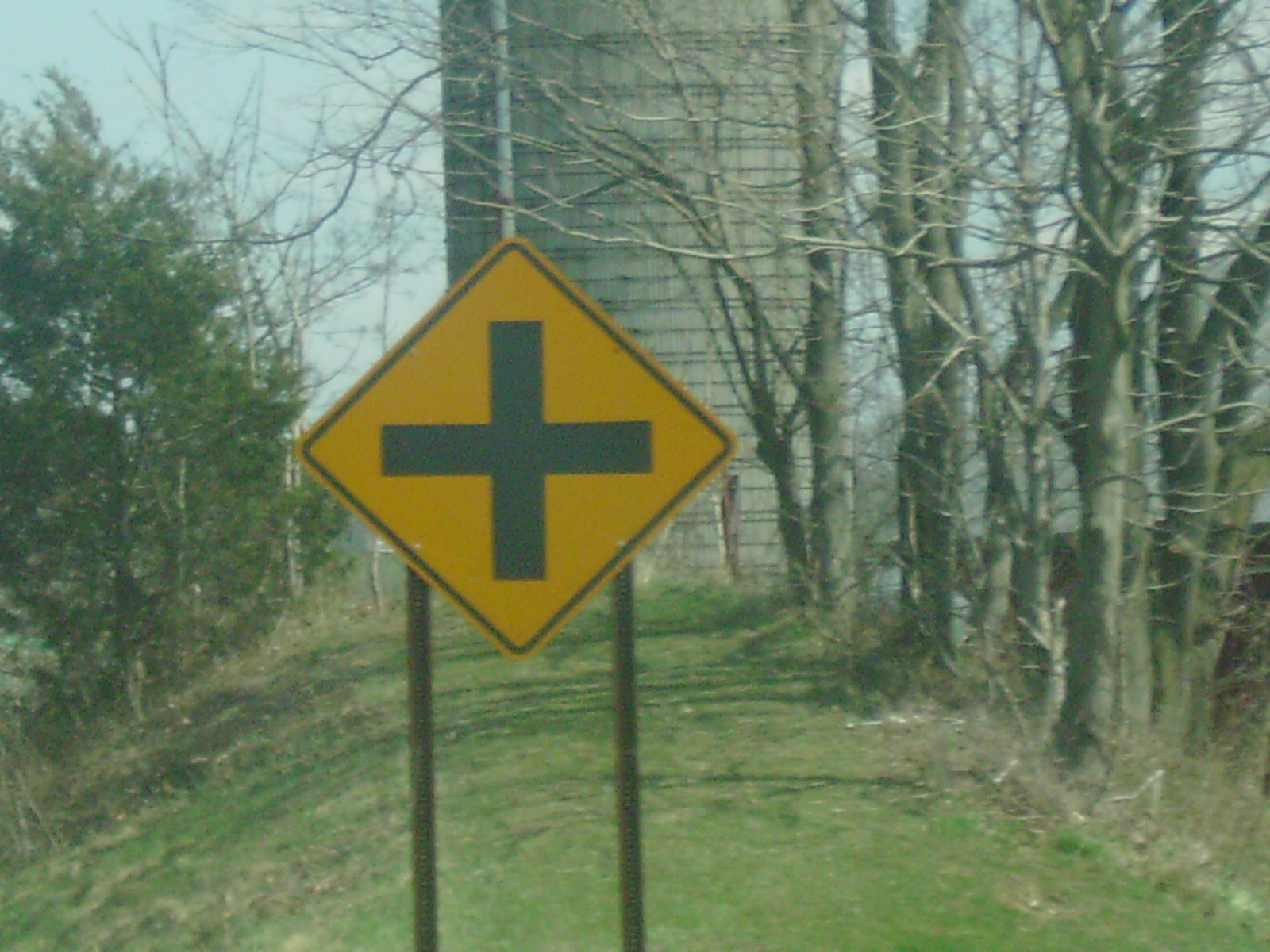This photograph captures a bright yellow, diamond-shaped road sign mounted on two rust-colored steel poles. The sign, featuring a bold black plus sign in its center, indicates a four-way intersection ahead. The sign stands on a grassy knoll with a backdrop of blue skies. To the left, there's a cluster of evergreen trees with green leaves, mingled with some bare birch trees. Behind the sign, a gray grain silo with a pipe running up its side is visible. On the right-hand side of the image, a line of leafless trees, their branches wild and intricate, adds a stark contrast to the greenery on the left.